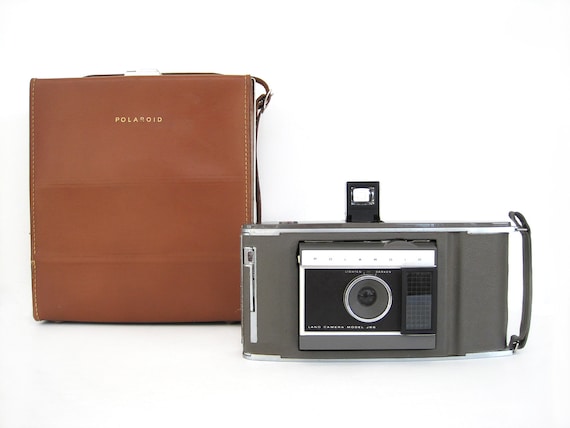The photograph captures a nostalgic scene featuring an old Polaroid camera accompanied by its brown leather carrying case. The leather case is situated on the left side of the image and is characterized by its rich brown color, detailed with white stitching along the edges and a zipper that runs along the top and side, though the precise configuration of the zipper is not fully discernible. The word "Polaroid" is tastefully embossed in small, goldish, possibly raised lettering on the case, which also includes a carrying strap attached with a metal clip.

To the right of the case stands the vintage Polaroid camera itself, distinctly gray with a more prominent black and white section in the center that houses the circular lens. The lens area is surrounded by a black panel featuring a small, grid-like pattern that resembles a solar panel. The flash unit is conspicuously extended from the top-center of the camera, black in color, and incorporates a small square viewfinder. A gray strap with silver metallic trim is affixed to the camera, enhancing its retro aesthetic. Overall, the image exudes a sense of historical charm, reminiscent of Polaroid's iconic 60s or 70s era.